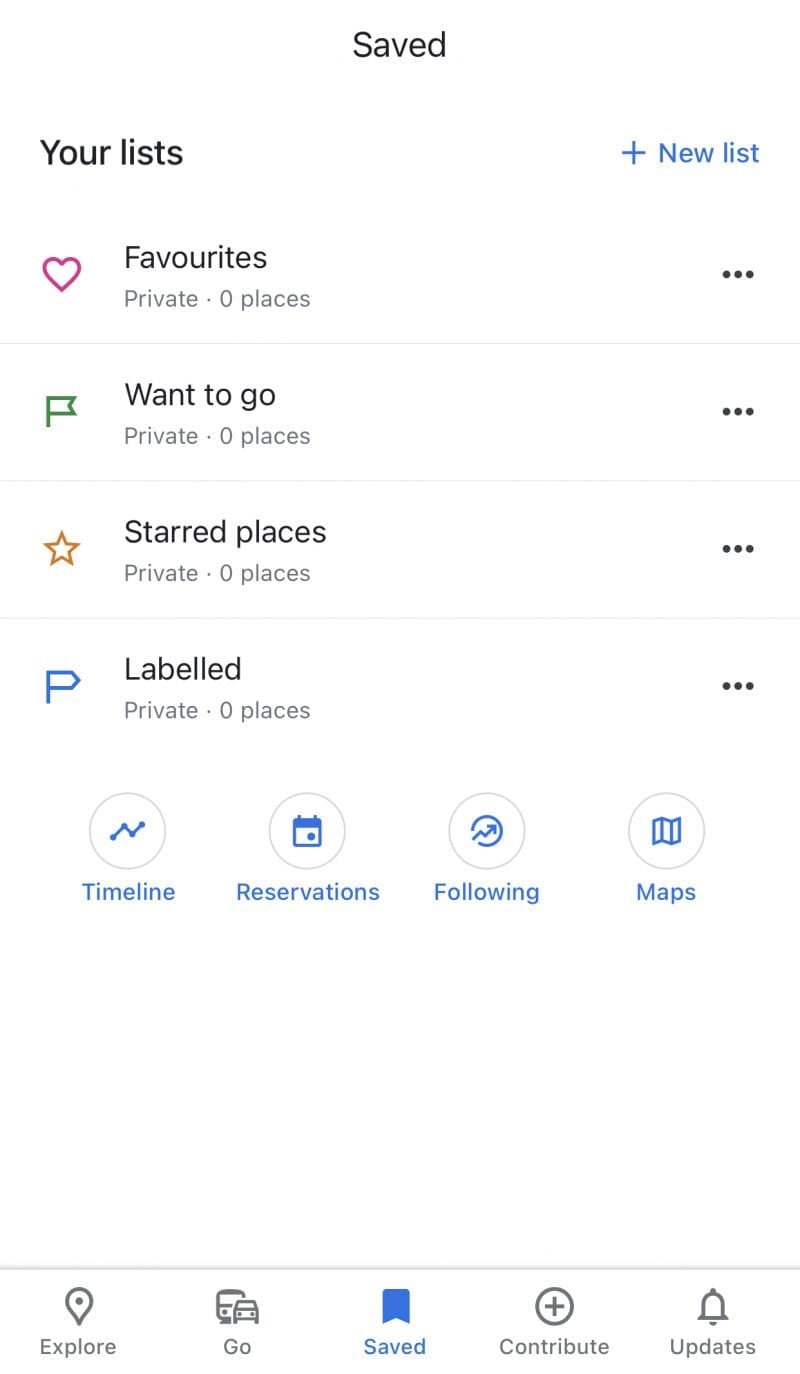The image depicts a user interface for a location-based application. At the very top center of the interface, the word "Saved" is prominently displayed. Below this, to the left, is the label "Your List" in black text, while to the far right, a blue text "New List" appears, accompanied by a plus symbol to its left.

Beneath "Your List," several categories are listed vertically: "Favorites," "Want to go," "Starred places," and "Labeled." Each category is marked as "private" and "places," with a count of zero nearby. Next to each category, distinct icons enhance visual identification: a pink heart for "Favorites," a green flag for "Want to go," a gold star for "Starred places," and a blue sign for "Labeled."

Further down the interface, three circular icons are aligned horizontally. The first, labeled "Timeline," is situated on the far left. To its right are "Reservations," "Following," and lastly, "Maps."

At the very bottom of the screen, five more navigation categories are indicated: "Explore" on the bottom left, followed by "Go," "Saved," "Contribute," and "Updates," neatly encapsulating the user’s potential activities within the app.